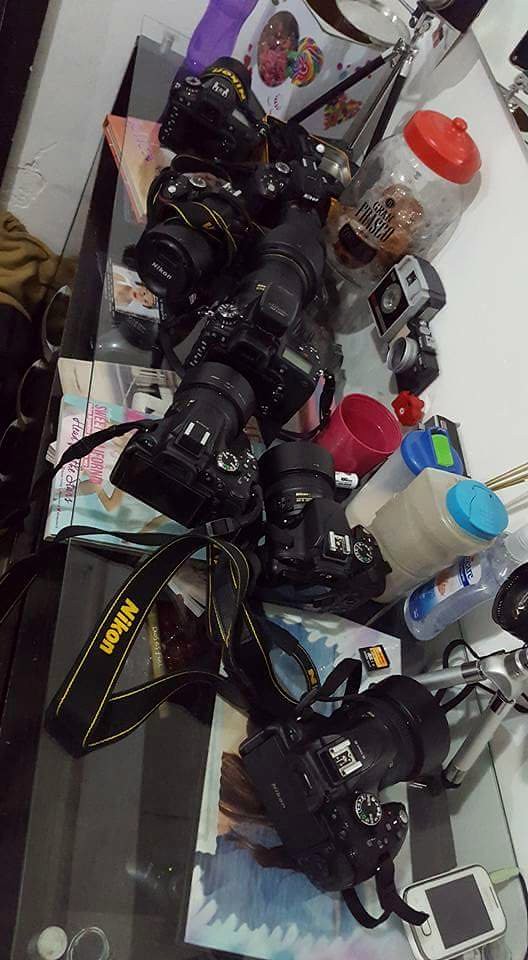In the image, there is a cluttered, multi-functional surface that resembles a bedside table or cabinet with a glass top layer elevated by short pillars above a brown base with drawers. The table stands against a white wall, likely within an indoor setting that might be an entryway or adjacent to a kitchen. A wide array of items cover the glass surface, highlighting its use as a catch-all for various household belongings. To the left, there's a purple cookie jar, followed by a black and silver tripod, and multiple cameras, including professional Nikon models with strap belts. Additionally, there are smaller cameras and camera chips scattered across. A red cup and a smaller pink cup, both containing water, are positioned centrally. Near these is a bottle that could be glycerine or clear baby oil. Towards the right side, there's another tripod and, further along, more cameras—counting up to a total of eight. On the far right bottom corner lies a small, older model white Samsung phone with a button, suggesting diverse technological device usage. Also visible are water bottles, likely a hand sanitizer bottle, and a jar with an orange lid that appears to contain candy. Amid the clutter, there seems to be a baby monitor screen, implying the presence of young children in the household.